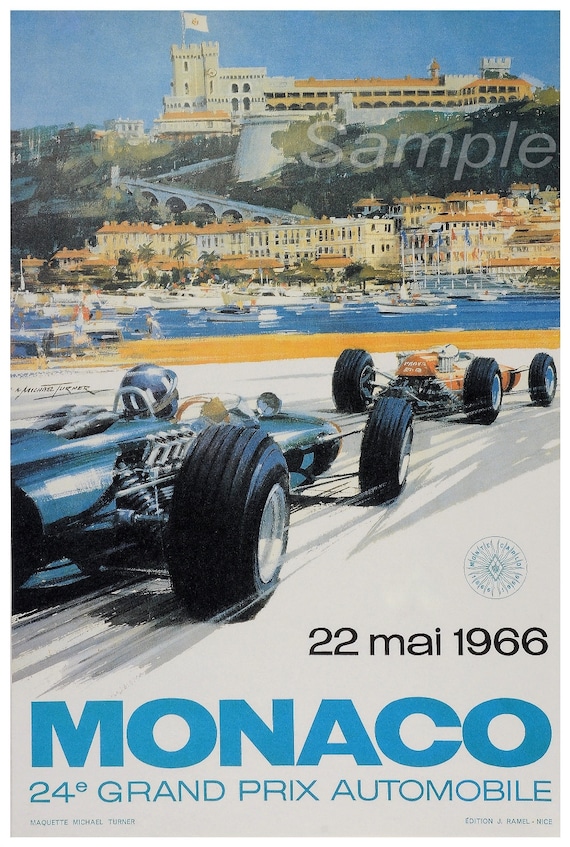This poster is an illustrated promotional piece for the "Monaco 24E Grand Prix Automobile," held on May 22, 1966. Rendered with stencils or colored pencils, the artwork showcases an exhilarating snapshot of the race. Two Grand Prix cars, one silver and one orange, speed down a light gray racetrack. The silver car, positioned slightly behind, features a single driver and a sleek, cigar-shaped design characteristic of the era. 

In the detailed background, a picturesque seaport city unfolds, revealing a marina filled with yachts and various high-rise buildings, presumably hotels and tourist complexes, along a pier. A hill adorned with a large castle, fort-like structures, and additional tall buildings rises on the distant horizon, contributing to the scene's depth and historical ambiance. 

The poster is marked by a "SAMPLE" watermark in white at the upper right corner and contains essential event details in both black and blue text at the bottom. Despite its vintage nature, the poster maintains a remarkable level of detail and vibrant quality, making it a captivating relic of motorsport history.